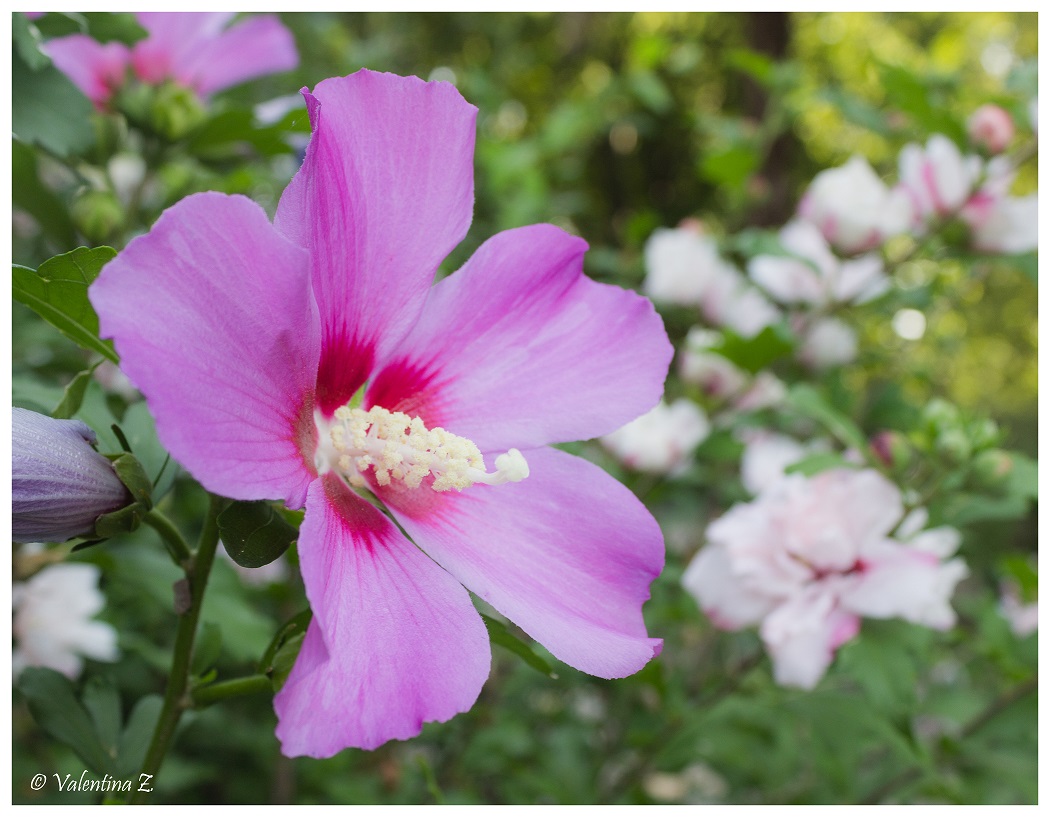This close-up image captures a stunning hibiscus flower positioned prominently towards the bottom left corner, slightly covering the center. The flower, featuring five delicate petals, displays a gradient from light pink to a purplish-pink hue, transitioning into a vibrant hot fuchsia pink at the core. Emerging from the center is a striking white stalk adorned with pollen, resembling a cluster of tiny cauliflower heads. The background showcases multiple hibiscus flowers, mostly in soft pink and white tones, with one flower yet to bloom near the upper left and a cluster of partially open flowers towards the lower right. The image is marked with a copyright for Valentina Z in white font at the bottom left-hand corner, adding a touch of artistic credit. The intricate details and vivid colors of the flowers create a captivating and dynamic composition.